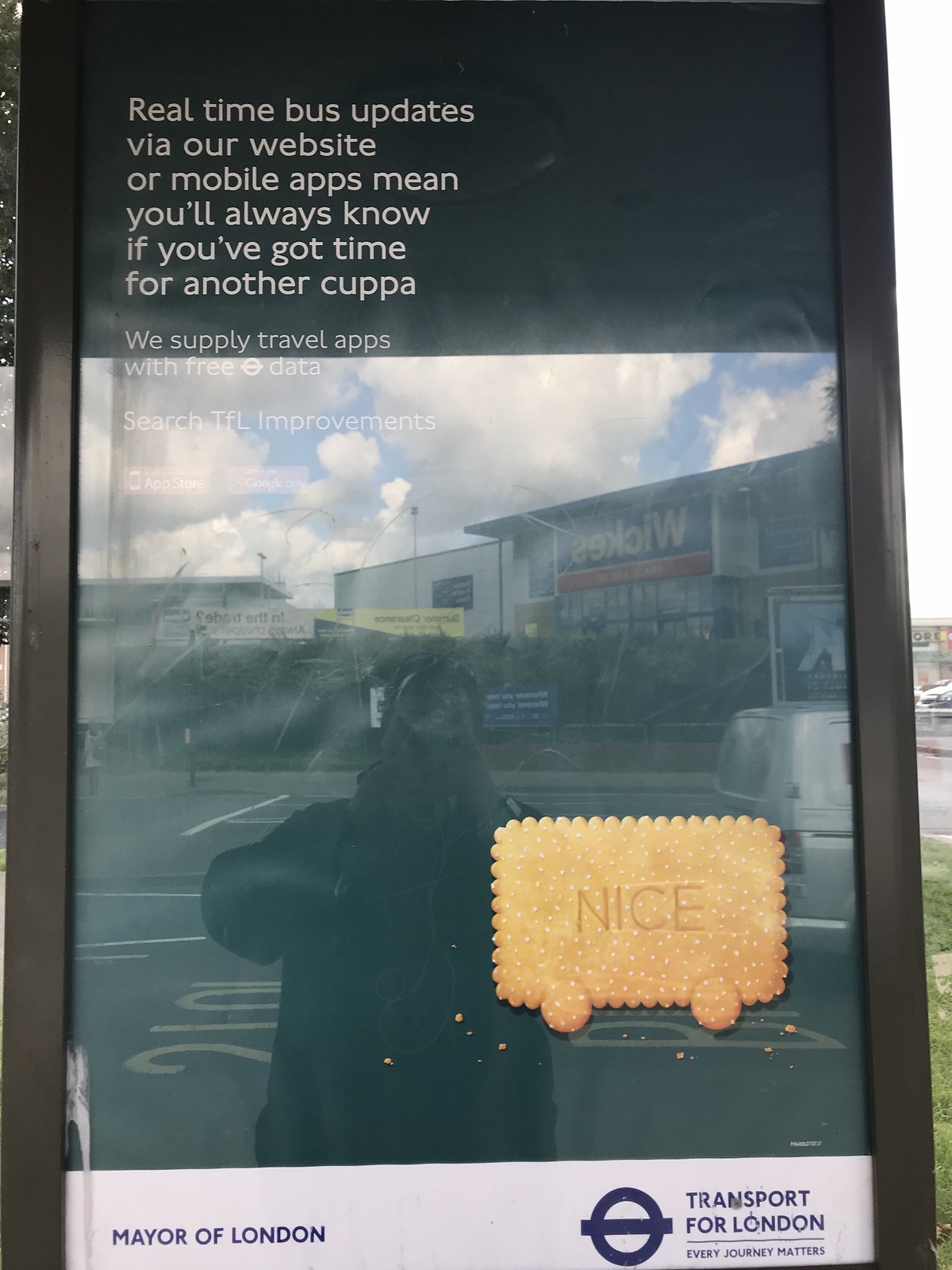This photograph, taken outdoors during a cloudy day, showcases a vertical bus stop sign encased in a reflective plexiglass cover, creating a vivid mirror-like effect that captures the photographer holding a camera, as well as the surrounding parking lot and buildings. The upper one-third of the sign has a black rectangular background with white text that reads, "Real-time bus updates via our website or mobile apps. Meaning you'll always know if you've got time for another cuppa." Below this, more text begins with, "We supply travel apps with free data, search TFL improvements," but becomes obscured by reflections. Toward the bottom of the sign, a white banner runs across from left to right, stating, "Mayor of London," and on the right, "Transport for London. Every journey matters." Adding a quirky touch, a sticker resembling a rectangular Ritz cracker with the word "nice" in its center and two small wheels underneath it is affixed above the Transport for London logo. In the reflective background, a silver van is parked to the right, and a building with a blue sign reading "Wicks" is visible, further enhancing the day's overcast ambiance.